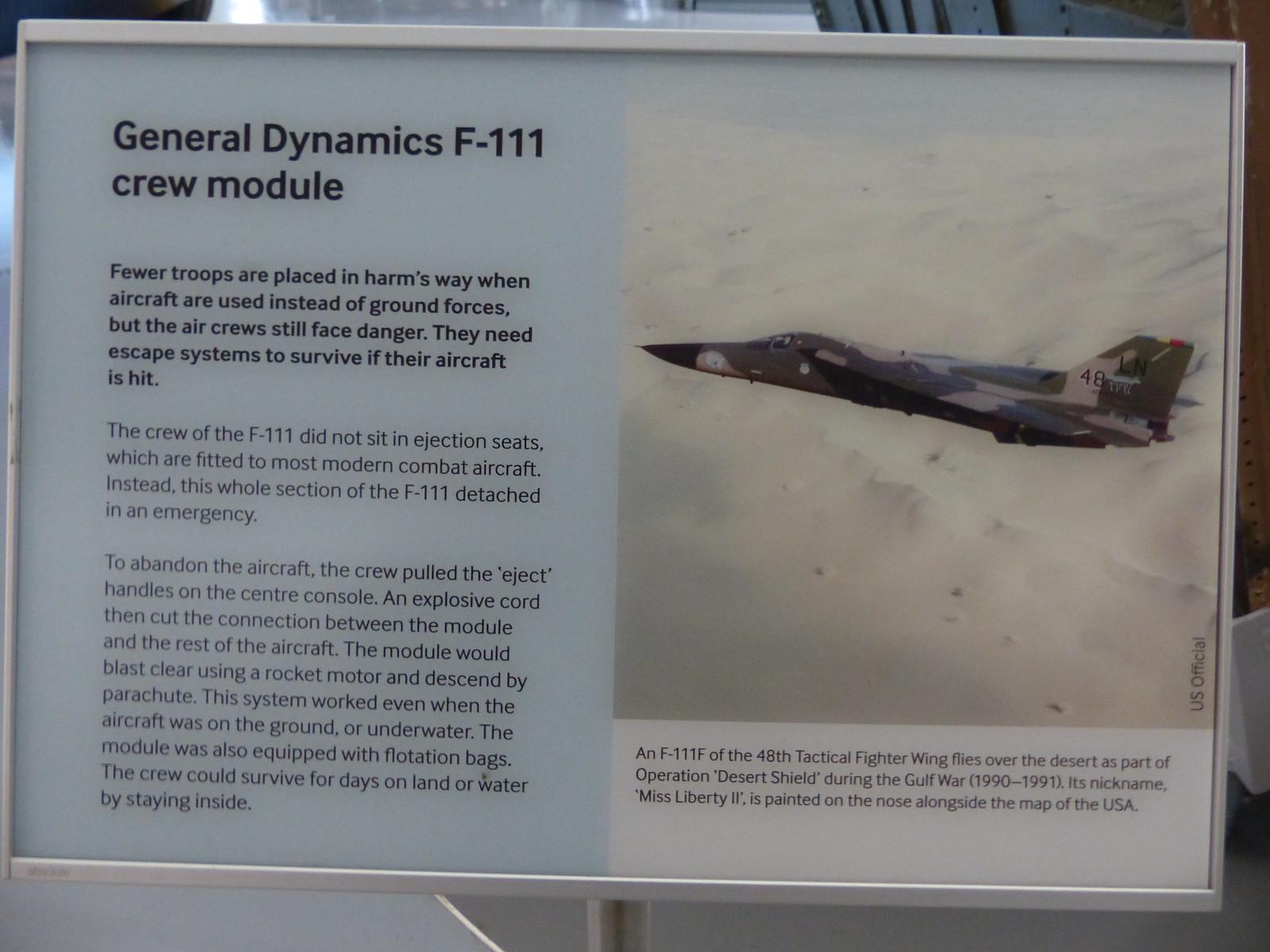The image is a close-up photograph of a museum display placard, which shows a slight tilt from a vertical plane. The placard is mounted on a pole visible at the bottom middle of the image. It primarily describes the General Dynamics F-111 Crew Module, prominently titled at the top. Below the title, a bolded paragraph explains that fewer troops are endangered when aircraft are used instead of ground forces, although air crews still face significant dangers and require effective escape systems.

The text elaborates that unlike most modern combat aircraft, which use ejection seats, the F-111’s entire crew module detaches during emergencies. To initiate this, the crew pulls eject handles located on the center console, triggering an explosive cord that separates the module from the plane. The module then blasts clear using a rocket motor and descends by parachute. Remarkably, this system functions even if the aircraft is on the ground or underwater. Additionally, the module is equipped with flotation bags, allowing the crew to survive for days on land or water by staying inside.

On the right side of the placard, there's a photograph of the military jet in flight over a desert landscape filled with sandy dunes. The jet features a camouflage pattern, blending into its arid surroundings. The environment slightly visible in the background of the image hints at the museum setting.